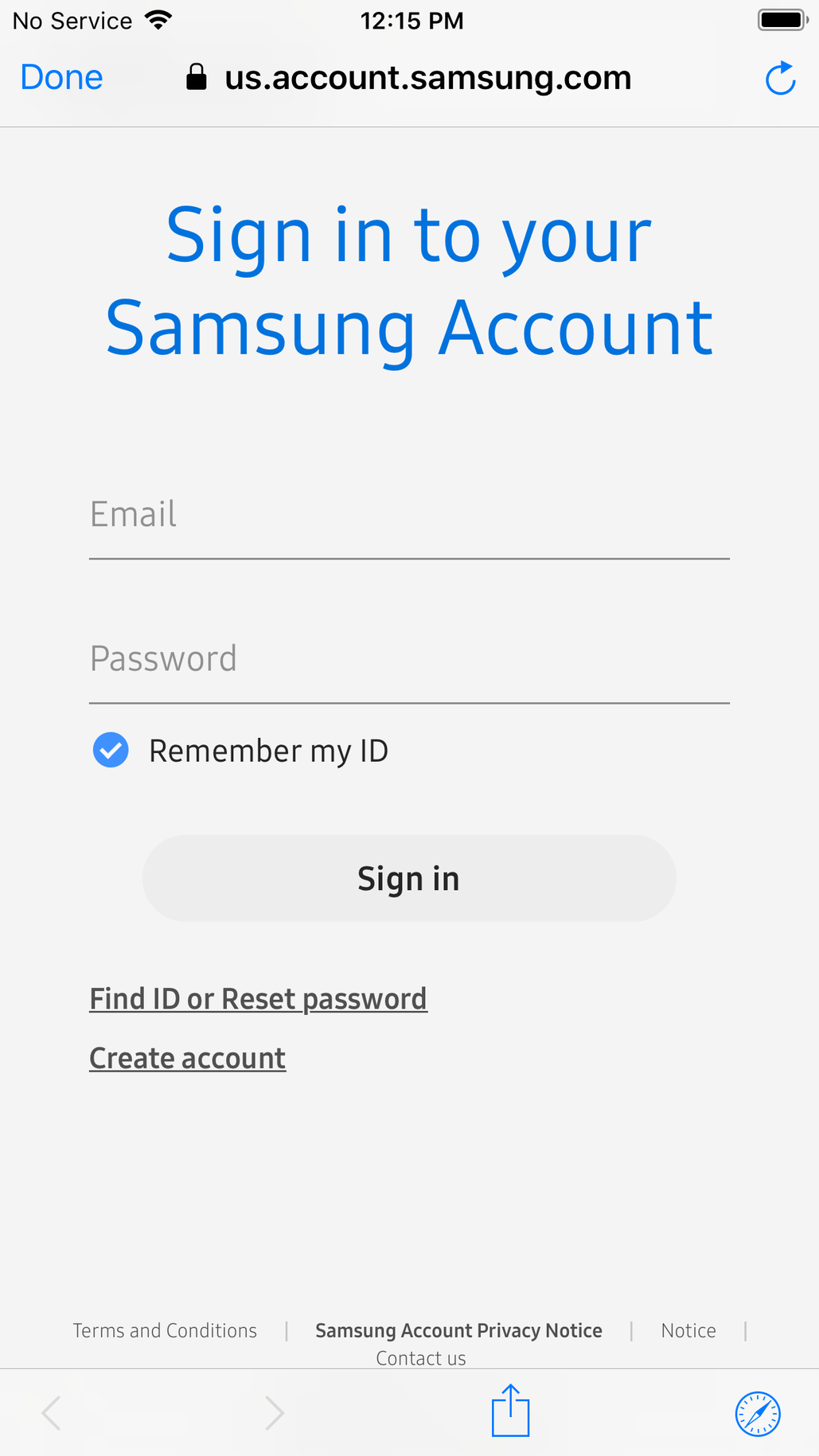The image displays a Samsung account sign-in page on a web browser. The page features a clean layout with a white background and blue text prominently displaying the message "Sign in to your Samsung account." Below this message are input fields for an email address and password, along with a checkbox labeled "Remember my ID." A blue "Sign In" button is shown for users to submit their credentials.

At the top of the page, the web address "us.account.samsung.com" is visible in the browser's URL bar. Adjacent to this, the browser interface displays a "done" button, indicates there is no network service, the time reads 12:15 PM, and the battery icon shows a full charge.

Directly under the sign-in fields, there are links for "Find ID or Reset Password" and "Create Account." The footer of the page contains further links to "Terms and Conditions," "Samsung Account Privacy Notice," and "Contact Us," followed by a couple of clickable blue icons.

In summary, this is a standard online sign-in page for Samsung accounts, visually straightforward and user-friendly.